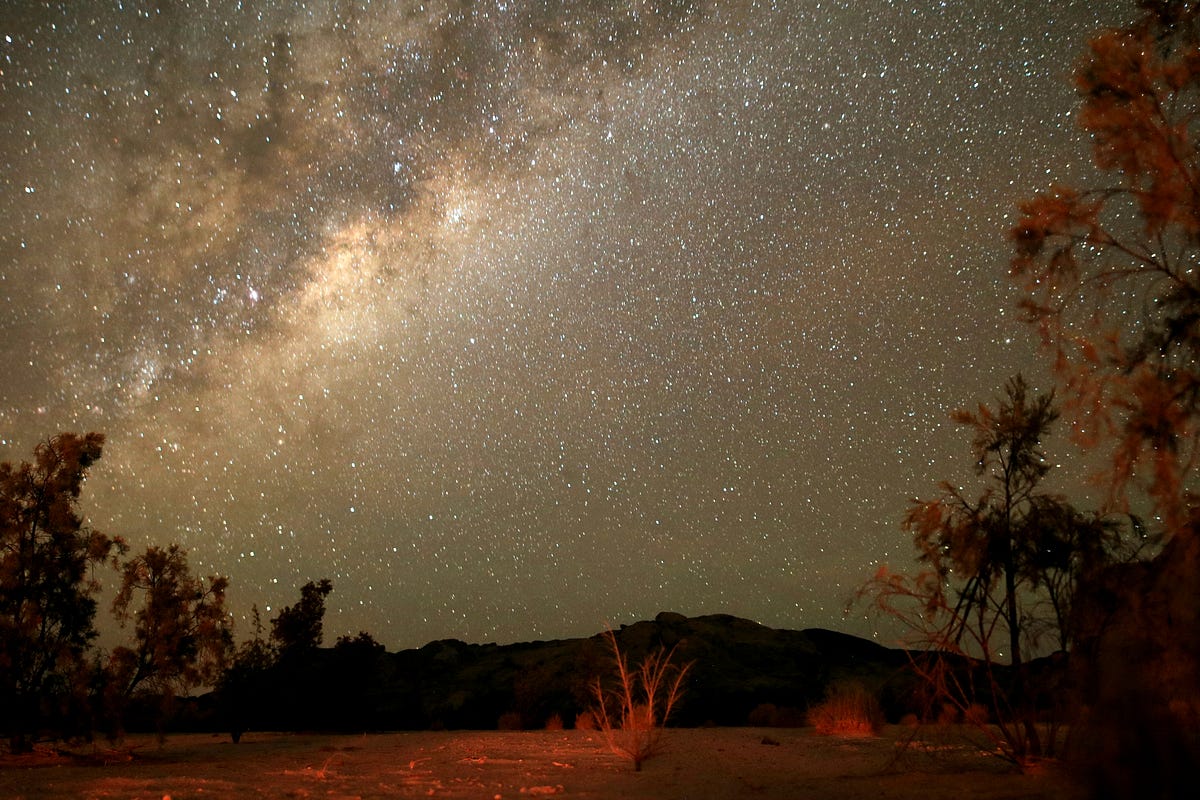This horizontally aligned rectangular image, possibly a painting or digitally generated picture, captures a serene nighttime scene dominated by a star-studded sky. The sky spans nearly the entire frame with a mesmerizing blend of browns, blacks, and grays, accented by hints of yellow and light brown near the upper left, where clouds obscure the moonlight. The myriad of bright, brilliant stars creates a breathtaking celestial canvas.

Beneath this expansive sky, a black, hilly terrain serves as a subtle divider. To the left, silhouetted trees fade into the darkness, while to the right, some trees display a mix of orange and darker green leaves, adding a touch of color to the night. The very bottom of the image features a brownish-red, glowing flat land, possibly illuminated by moonlight, with a lone bush or scrub brush growing out of it. This enchanting scene captures the tranquility of a remote, unlit landscape under a stunning night sky.